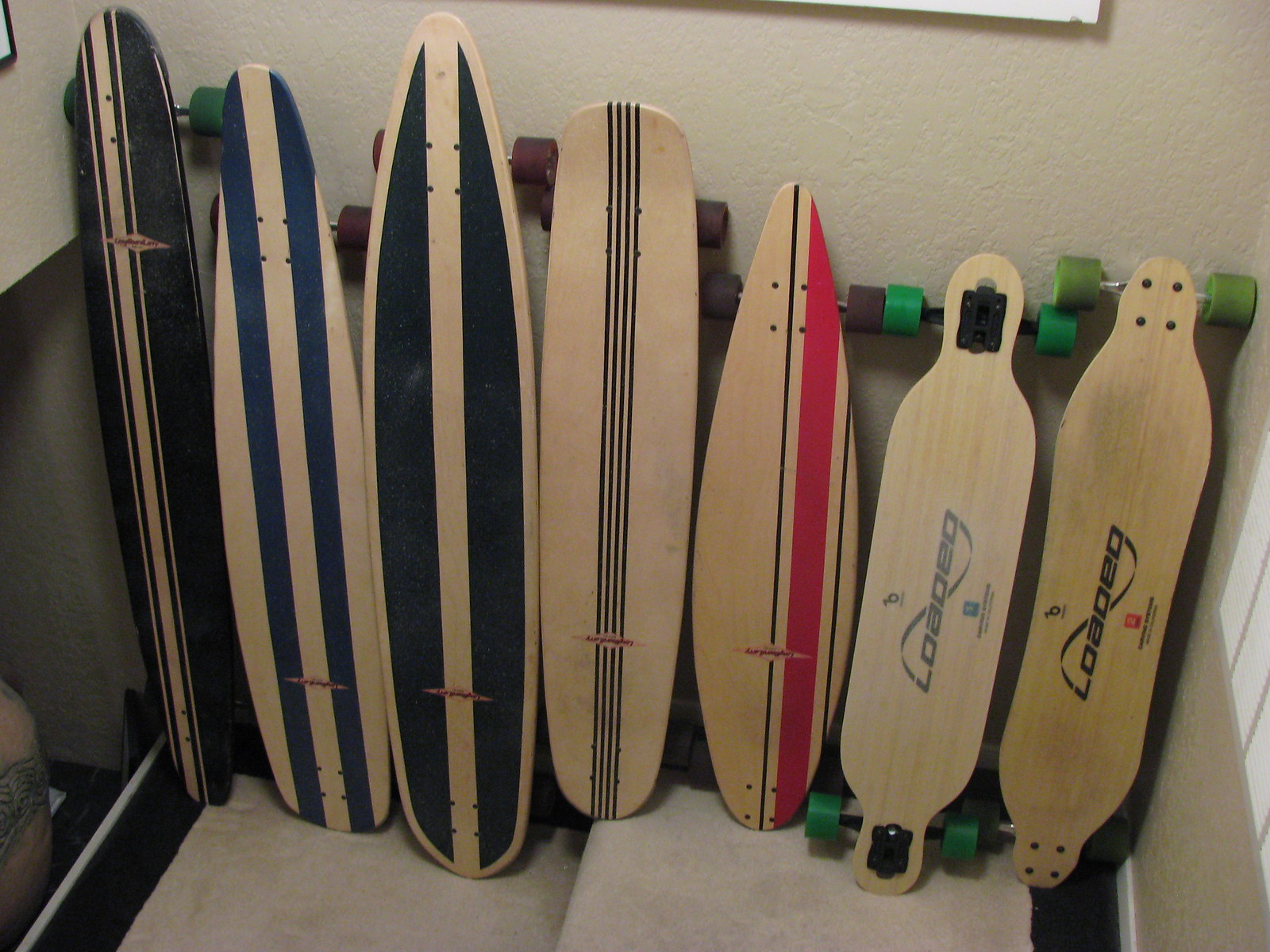This photograph captures an assortment of seven skateboards and longboards leaning against white walls in what seems to be a small enclosed space, possibly a closet or cubby area. The boards are arranged from left to right, starting with the longest on the left and progressively getting shorter towards the right. The boards have a tan birch material with multiple decorative features. 

The first board on the left has red wheels, while the rest of the boards on the left side, including the large black one with two vertical lighter wood strips and a shallow diamond-shaped logo, also carry unique designs. The second board has two vertical black strips, and the third one displays similar black inlays. The fourth board features a wooden top decorated with three or four black pinstripes. The fifth board resembles a bowling pin with a central red stripe flanked by thin black pinstripes.

Moving to the right side, the last two boards are notably shorter and bear the logo "Loaded," with wide trucks and green wheels. These 'Loaded' boards feature a ribbon-like branding and cutaway sections that make them narrower near the trucks. Despite their differences, none of the boards appear to have the conventional grip tape.

The color palette in the space includes the white of the walls, the brown of the carpeted floor, and the tan, black, blue, and red accents on the skateboards. The arrangement and the distinctive details present a visually engaging display of longboarding and skateboarding gear.